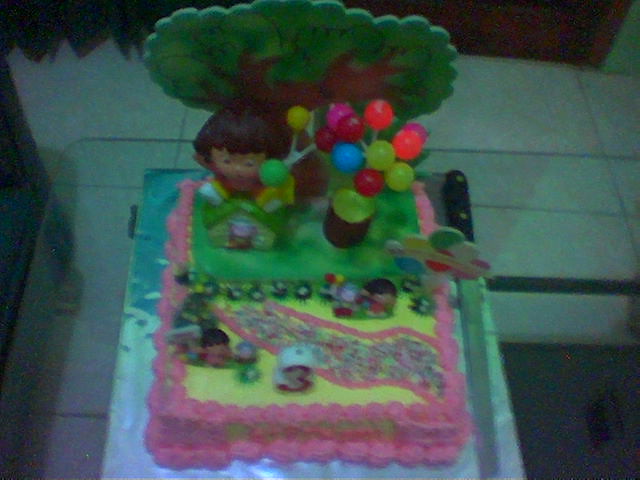The image depicts a rectangular Dora the Explorer-themed birthday cake for a three-year-old child, viewed from above. The surface of the cake is designed to resemble a grassy scene, with Dora the Explorer sitting with her arms raised and short brown hair, positioned in front of a large cardboard or foam board cutout of a tree. Next to Dora is a dark black cylindrical pot-like object filled with multicolored lollipops that resemble balloons. A bubblegum pink icing trim outlines the cake, while a pink and multicolored pathway traverses a section of the cake's yellow frosting. Prominently located in the center is a candle shaped like the number three. The cake sits on a silver tray, which is placed on a table. To the right of the cake, there is a long knife with a silver blade and a brown handle. The background includes what appears to be white square tiles and some indistinct brown and gray objects.